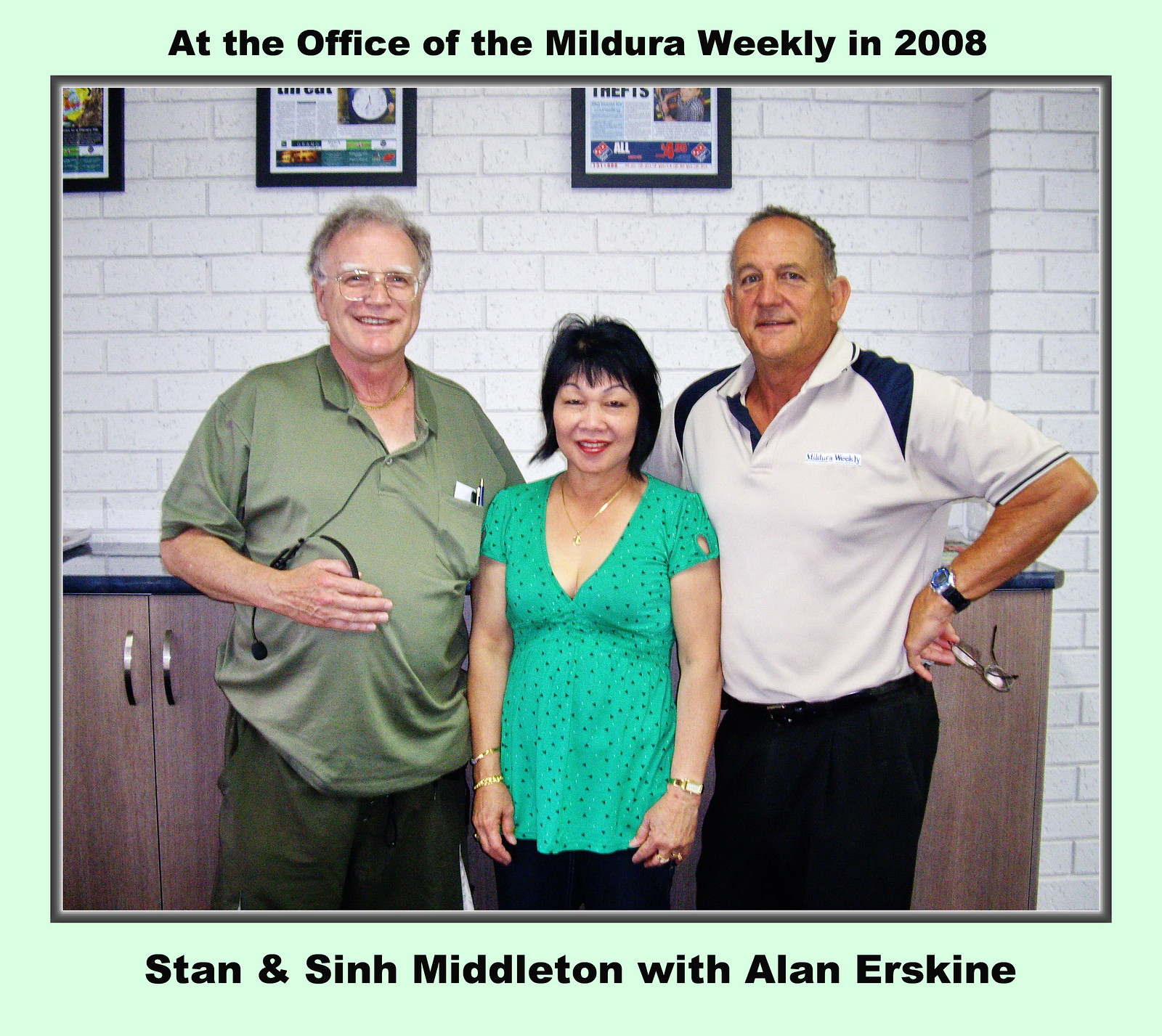This photograph, taken indoors at the office of the Mildura Weekly in 2008, is framed by a thin gray border and a larger mint green border. Encased within this frame, a black print caption reads "At the office of the Mildura Weekly in 2008" at the top, and "Stan and Sinh Middleton with Alan Erskine" at the bottom. The image itself captures three people standing against a white brick wall, with a wooden cabinet and parts of a few framed pictures in the background.

In the center stands Sinh Middleton, a small, older Asian woman with slightly spiky, straight black hair and bangs. She is smiling directly at the camera, showcasing her upper teeth accentuated by red lipstick. She is dressed in a short-sleeved, green tunic with black polka dots featuring a v-neck and a gold necklace.

To Sinh's left is Stan Middleton, an older man with pale skin, gray hair, and wire-framed glasses. He has a slightly heavyset build with a pot belly and is dressed in a green polo shirt and darker olive pants. He stands with his left arm bent at the elbow, his hand in front of his stomach with fingers together, sporting a smile that lifts a bit higher on the left side.

On Sinh's right is Alan Erskine, who appears to be around 62 years old with short, gray hair and slightly tanned skin. He is wearing a cream-colored golf shirt with navy accents on the shoulders and navy stripes at the end of the sleeves, paired with black pants. His left hand holds a pair of glasses, adorned with a navy and silver watch, while his right hand rests behind Sinh. The shirt features the "Mildura Weekly" logo on it, subtly highlighting their workplace connection.